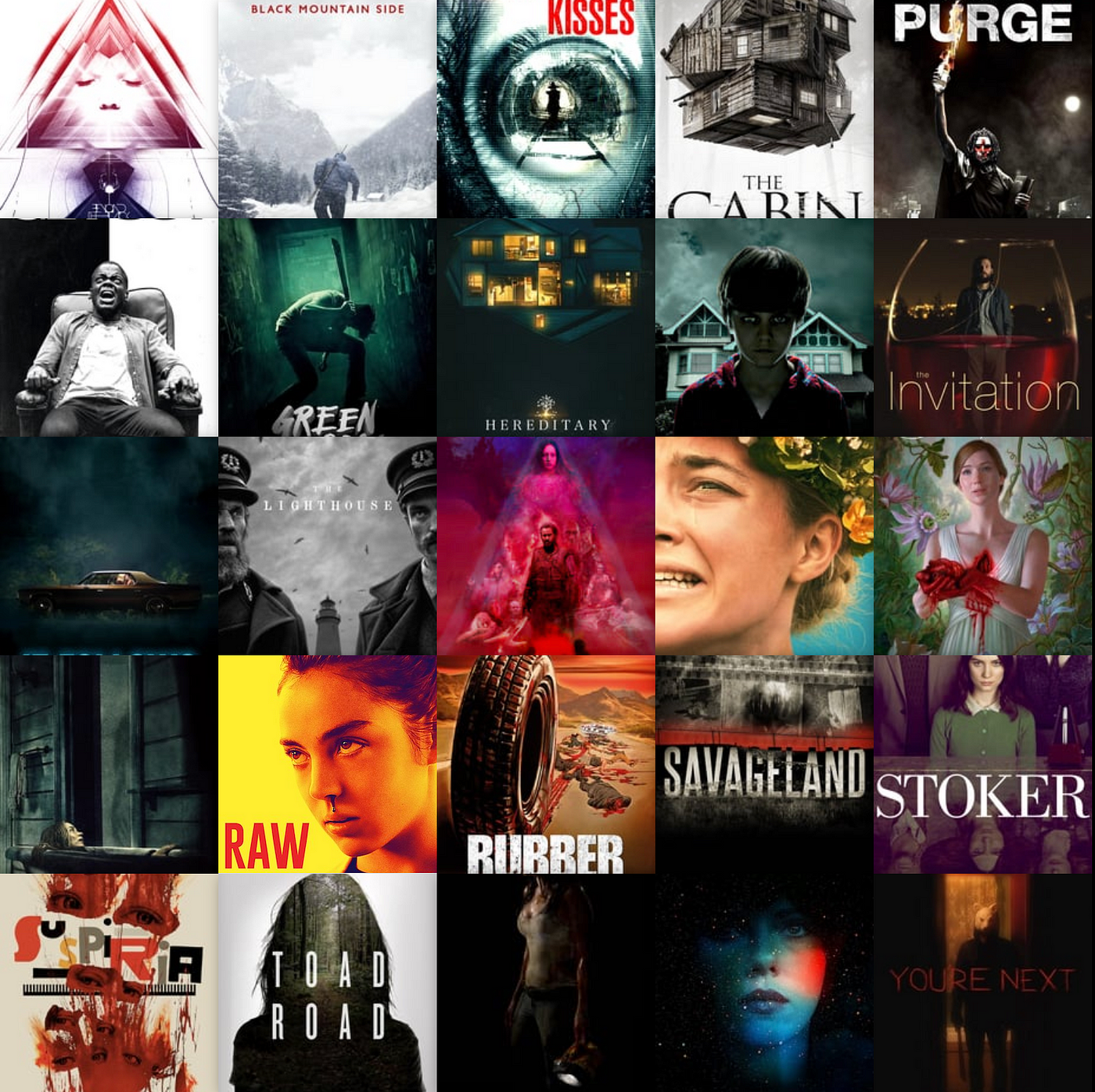The image is a 5x5 grid comprising 25 movie posters, heavily leaning towards the horror and thriller genres. Starting from the top left, the first poster features a face within a triangle. Next is "Black Mountain Side," showcasing a man walking in a black-and-white mountain scene. "Kisses" displays a person in a tunnel with red text, followed by "The Cabin" with a cabin image against a white background. "The Purge" presents a figure holding a Molotov cocktail. 

The second row begins with an image of a person screaming in a chair, followed by the green-hued "Green" poster. "Hereditary" shows a two-story house brightly lit from within, and "The Invitation" features a kid with an outlined eye and a menacing house in the background.

The third row includes "The Lighthouse," with an uncertain dark scene, and a pink-colored poster recognized as "Midsommar," though not labeled. Another poster shows a woman in a garden holding a bloody heart.

The fourth row begins with a non-identifiable dark poster, "Raw" with a woman sporting a bloody nose, "Rubber" showcasing a giant tire, "Savage Land," and "Stoker."

The final row includes a poster for "Suspiria" with an abstract design, "Toad Road" featuring a dark figure, and three largely indistinguishable dark posters. Other notable mentions within the grid are "You're Next," "Stoker," and "Savage Land," contributing to the overall eerie and spooky atmosphere of the photo.